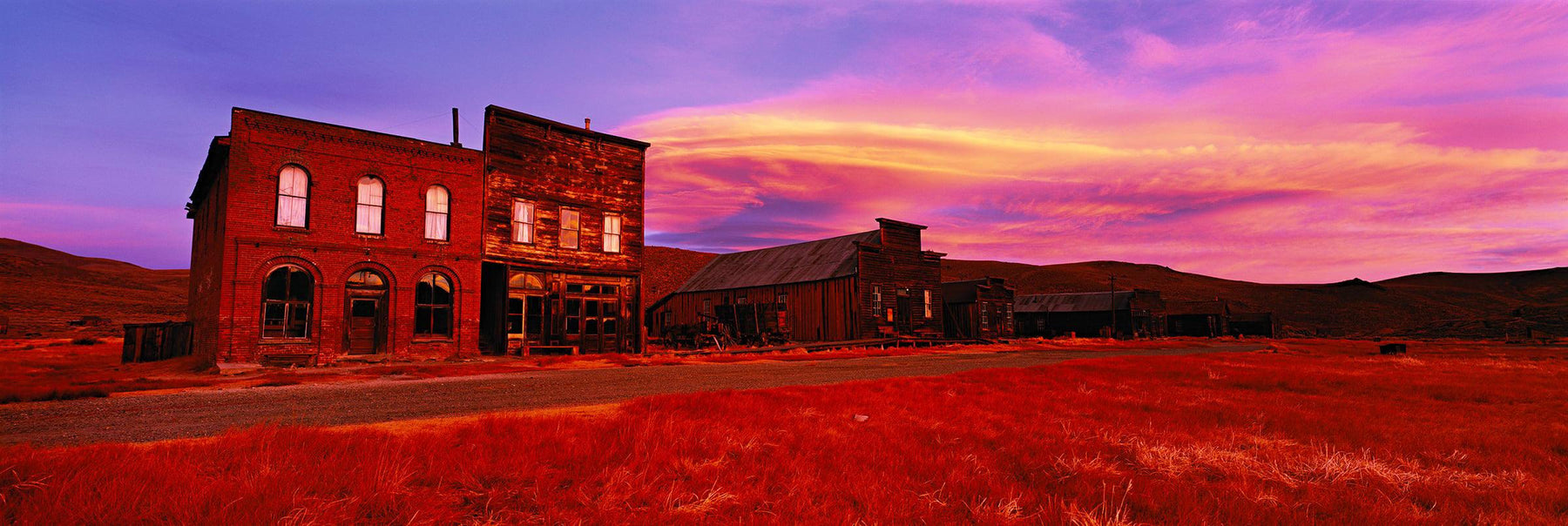This panoramic photograph captures a vivid, breathtaking sunset with colors ranging from blue and purple to pink, orange, and yellow, scattered across a cloud-streaked sky. The image, a wide rectangular shot with the long sides at the top and bottom, portrays an old, seemingly abandoned town nestled in a hilly, mountainous landscape. In the foreground, a dirt road winds through dead, hay-like grassy fields. The town consists of several run-down, wooden buildings with broken windows and doors, presenting a mixture of residential and commercial architectural styles, reminiscent of an old 1800s desert town. The forefront features two prominent two-story structures with large windows, their reddish hue possibly accentuated by a photographic filter. Further into the distance stands a weather-beaten, long cabin-style building, indicative of commercial or industrial use, with its long wall mostly collapsed. The ensemble of decayed structures extends into the background, adding depth and a haunting beauty to the striking scene.